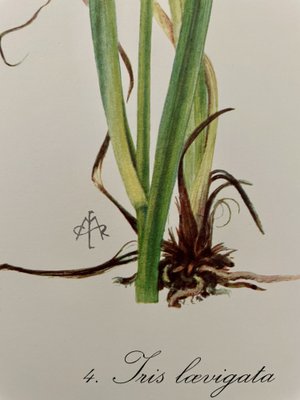This image is a detailed botanical illustration or watercolor painting on a white background, depicting a green plant with an intricate root system. The central focus is on the green stems, which branch out and are accompanied by partial leaves. At the base, the plant's root system is shown with brown tendrils and lighter brown roots extending outward. The image is labeled with "Iris laevigata," marking it as a depiction of this particular iris species. The number four is positioned at the bottom of the page, suggesting it could be part of a series. The artist's signature appears to be a pictogram resembling an A intertwined with an R. This artwork is reminiscent of traditional naturalist illustrations typically found in herbariums.